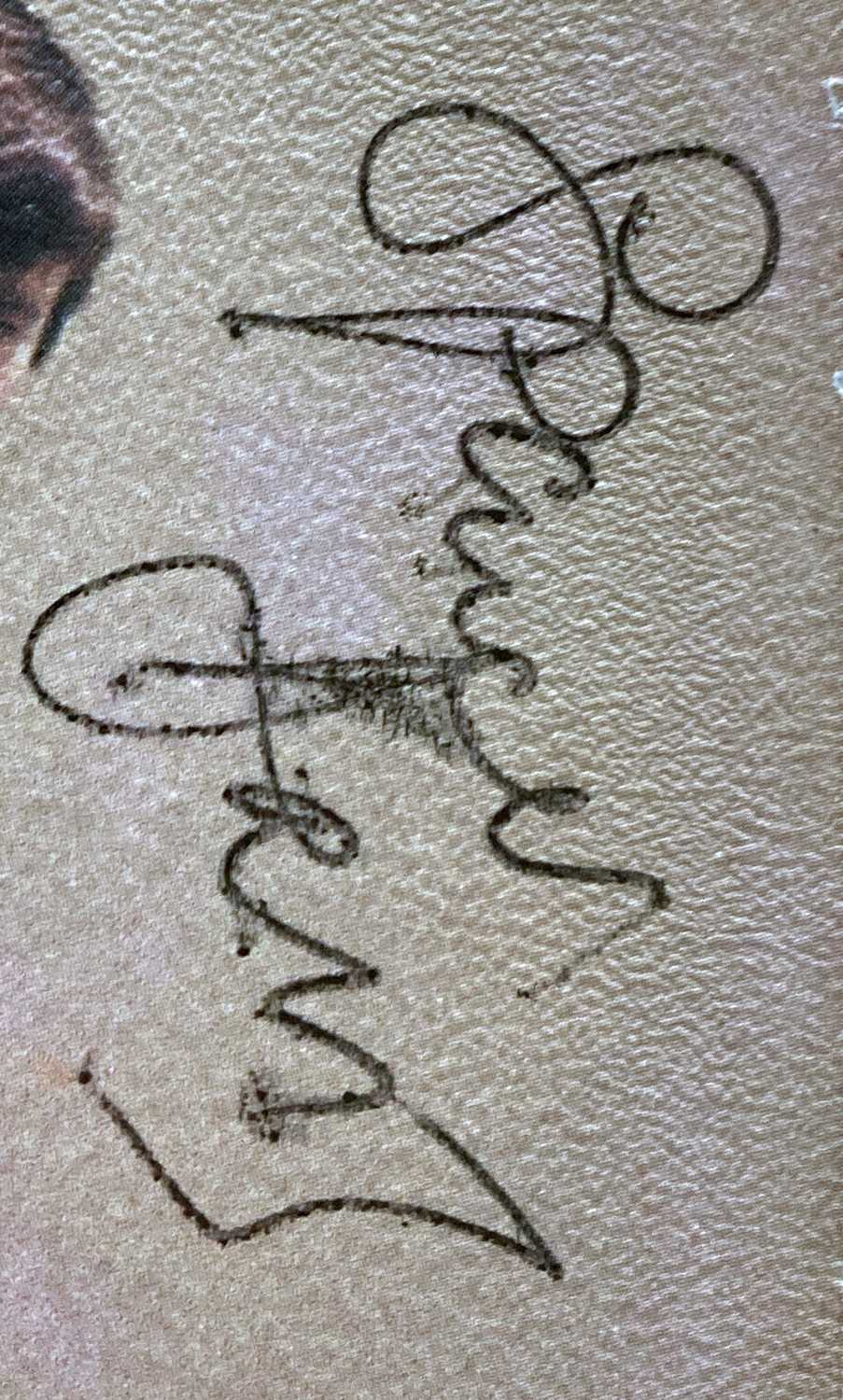The image displays the intricately crafted signature of Spencer Jones, the center fielder for the New York Yankees. The autograph is executed in black ink, likely from a thin black magic marker or pen, on a textured, white surface resembling plaster with a bumpy texture and small bubbles. The signature is oriented vertically, requiring a 90-degree rotation to the left to read properly. The first name, "Spencer," is clearly legible, with a distinct decorative 'S' and all letters spelled out. The last name appears as "J-O-N," followed by a sweeping end that resembles an 'S' or a 'Z'. In the bottom left-hand corner of the photo, there's a partial glimpse of the person writing it, showing a bit of hair and the forehead, or possibly an animal with brown and white fur.